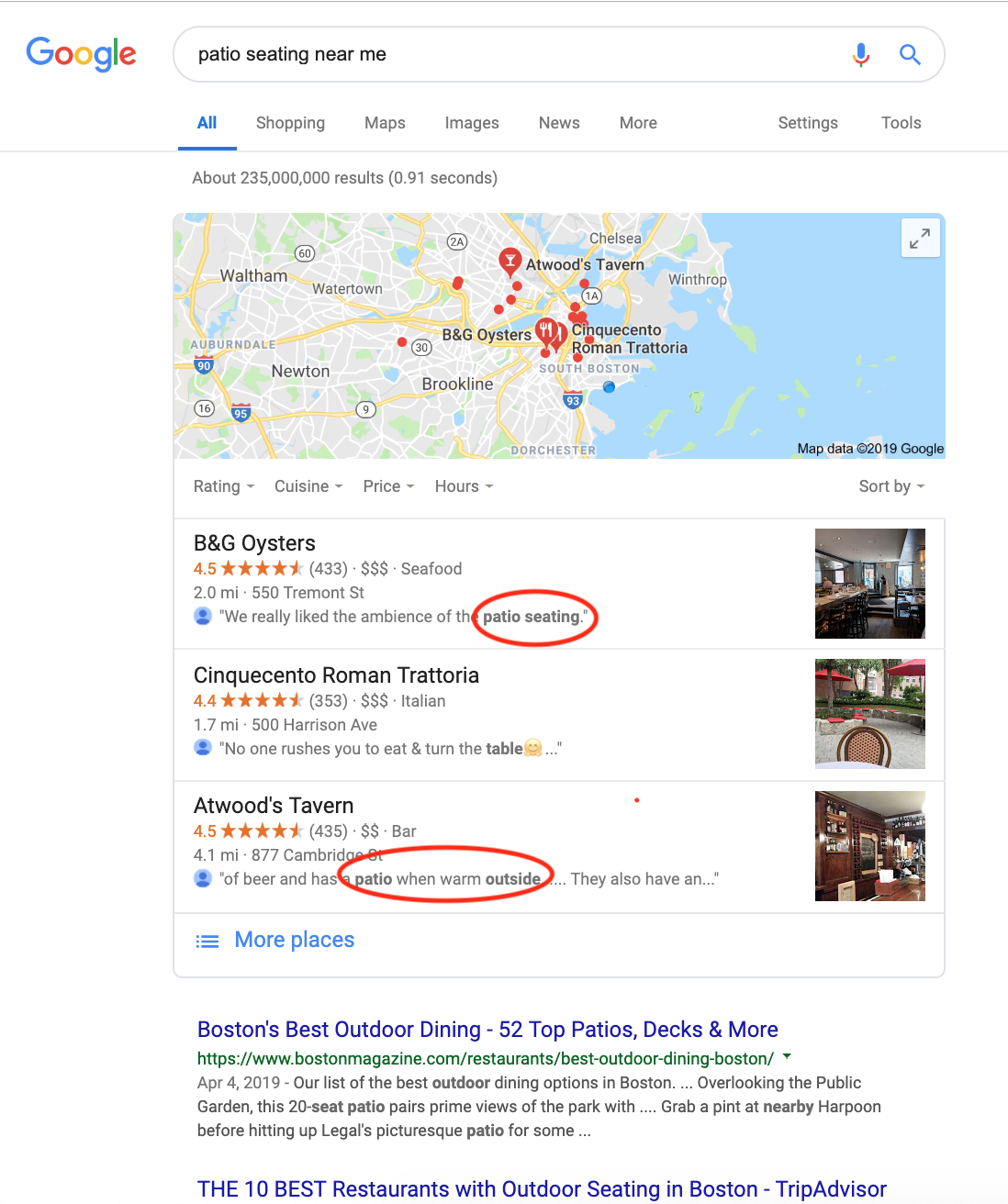In the image, we are viewing a Google Maps interface. In the top left corner, the Google logo is prominently displayed, featuring the familiar blue "G," red "O," yellow "O," blue "G," green "L," and red "E." Adjacent to the logo, there is a search bar with the query "patio seating near me."

Below the search bar, there are filter options highlighted in blue. The map displayed focuses on the Boston area, marked with red dots indicating various locations, and shows a network of roads and cities. Noteworthy landmarks include a body of water adjacent to the city area.

Highlighted on the map are three restaurants relevant to the search:

1. **B&G Oysters** - Rated 4.5 stars, located 2 miles from the search origin. The option for patio seating is circled in red.
  
2. **Cinquecento Roman Trattoria** - Rated 4.4 stars, not specifically marked for patio seating.
  
3. **Atwood's Tavern** - Rated 4.5 stars, located 4.1 miles from the search origin. The map notes that patio seating is available when the weather is warm, marked with a red circle.

Below the map, there is an additional search suggestion titled "Boston's Best Outdoor Dining" with a link to "52 top patios, decks, and more." This provides further options for outdoor dining in the area.